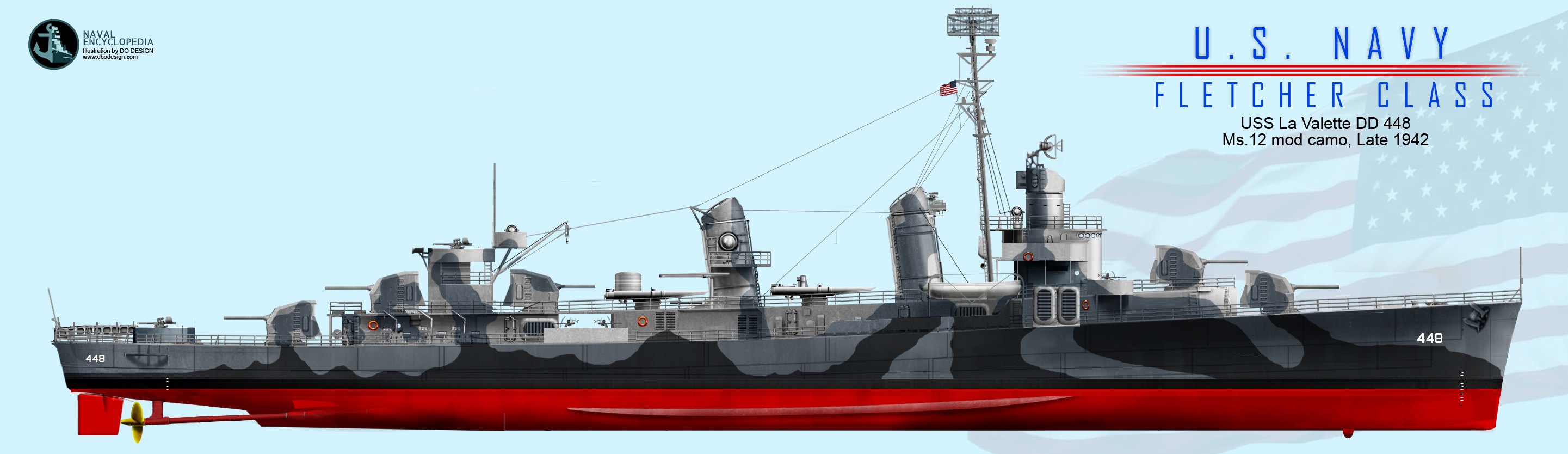This digitally created illustration showcases the USS Lavalette (DD-448), a Fletcher-class destroyer of the US Navy from late 1942, set against a light blue background. Dominating the center is the intricately detailed ship, which features a distinct color scheme: its hull is primarily gray with darker gray lines, and it is set off by a thick red horizontal stripe at the bottom. The image captures essential Navy characteristics such as multiple large turret guns, various mounted smaller guns, and a small US flag. 

In the upper right-hand corner, prominent blue text reads "U.S. Navy," followed by four red horizontal lines. Beneath, in blue, the words "Fletcher Class" are displayed, with further details in black text stating "USS Lavalette DD-448, MS-12 Mod Camo, late 1942." The upper left corner houses a Naval Encyclopedia logo—a black circle containing a light green anchor—accompanied by small, hard-to-read text. The overall composition, intended for educational and informational purposes, balances professional graphic design with historical accuracy, ideal for web pages or informational resources.